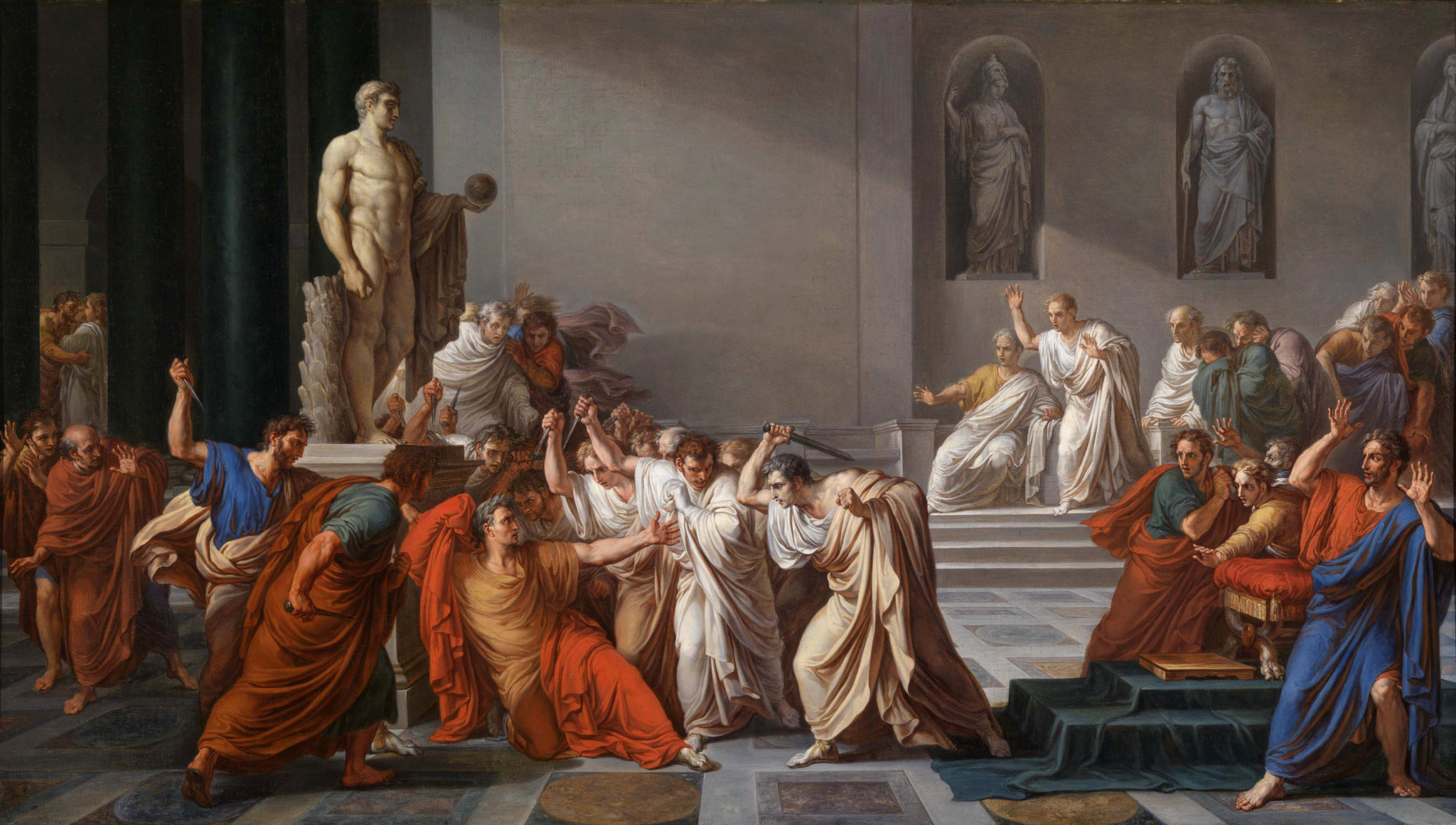The painting is an elaborate, realistic depiction seemingly set in Roman times, reminiscent of the assassination of Julius Caesar. It captures a dramatic scene inside a stately palace adorned with various large Roman statues, including a prominent nude figure in the background. The central figure, a man who appears to be falling or lying on the floor, is surrounded by a mix of men in different colored robes—red, white, green, blue, and yellow. Some of these men brandish knives, poised to strike, while others lean away in shock or fear. The expressions and stances of the men suggest a chaotic and violent moment, with some attacking the central figure and others attempting to protect him. The tension in the scene is palpable, as the surrounding men either join in the violence or recoil in terror, capturing the intensity and turmoil of a significant historical or dramatic event.